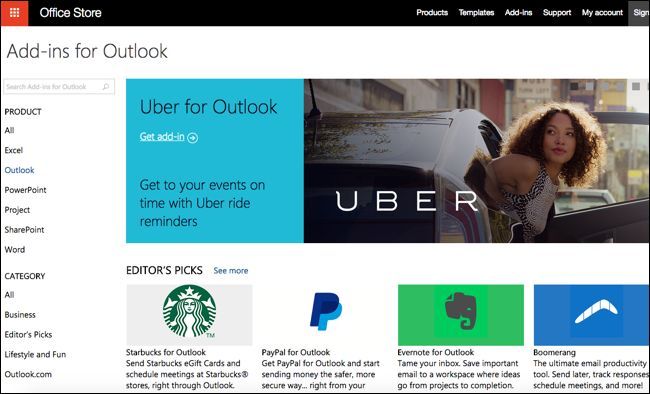**Detailed Caption:**

The image depicts the home page of a store named "Office Store." The store's title is displayed at the very top left corner on a black banner with white text. At the top right corner, there is a logo composed of nine dots arranged in a grid pattern against a red background. Adjacent to this logo, aligned from left to right, are the navigation menu items: "Products," "Templates," "Add-ins," "Support," "My Account," and "Sign-in," although the end of the "Sign-in" text is slightly cropped out.

Below the main navigation, towards the left, there is a header that reads "Add-ins for Outlook." A prominent banner features a woman, possibly biracial and light-skinned, with curly hair stepping out of a black car. She is looking upwards to the left, and the word "Uber" is prominently displayed to her left in white text. Next to the woman on the left side, there is a teal square containing the text: "Uber for Outlook, get add-in." Below this, a subtitle reads: "Get to your events on time with Uber ride reminders."

To the far left of the page, a vertical list categorizes the content. The categories under "Product" include: "All," "Excel," "Outlook," "PowerPoint," "Project," "SharePoint," and "Word." Below that, the categories under "Category" include: "All," "Business," "Editor's Picks," "Lifestyle and Fun," and "Outlook.com." 

Next to this list is a section titled "Editor's Picks" with a link to "See more." Below this, several logos are displayed, each accompanied by a descriptor. These logos include: the Starbucks logo with a white background and green siren, the PayPal logo featuring two 'P's, one dark blue and one light blue, the Evernote logo represented by a side profile of a cartoon elephant in gray against a green background, and the Boomerang logo which depicts a boomerang in an upside-down 'V' shape on a blue background. Correspondingly, the text next to these logos reads: "Starbucks for Outlook," "PayPal for Outlook," "Evernote for Outlook," and finally "Boomerang."

The entire layout is set against a clean, white background.